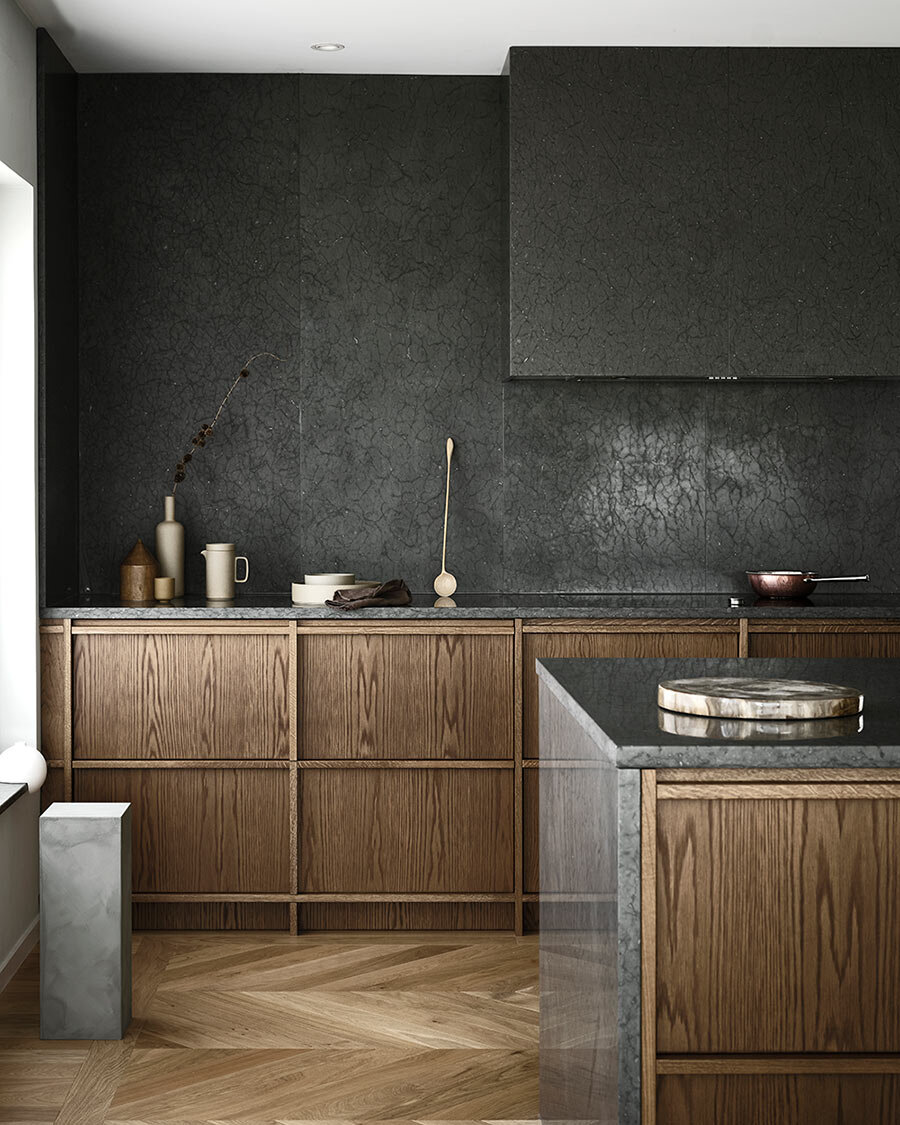The image shows a designer kitchen with a modern, sophisticated aesthetic. Central to the composition is a dark gray paneled wall and cabinetry that creates a sleek backdrop, complemented by a charcoal gray marble countertop. The wooden lower cabinets exhibit a medium brown hue with a crossboard design, and intriguingly lack visible handles, suggesting a minimalist touch or hidden mechanisms.

Upon the marble countertop, several objects are meticulously arranged. A notable item is a creatively repurposed wine bottle, painted white, acting as a narrow vase with dried flowers artistically protruding from the top. Next to it sits a pitcher likely intended for water, its design harmonizing with the ambient palette. Near the pitcher, a shining copper pan with a metal handle catches the eye.

A stainless steel disc adorns the front island, enhancing the sleek, utilitarian appeal of the kitchen. The wall above the countertop has a contrasting finish that resembles suede, contributing to the room’s textural depth. A window to the left edges the scene with natural light, adding a subtle, inviting warmth. Without visible sinks or stoves, the image focuses on the kitchen's design and the sophisticated, thoughtful arrangement of its elements.